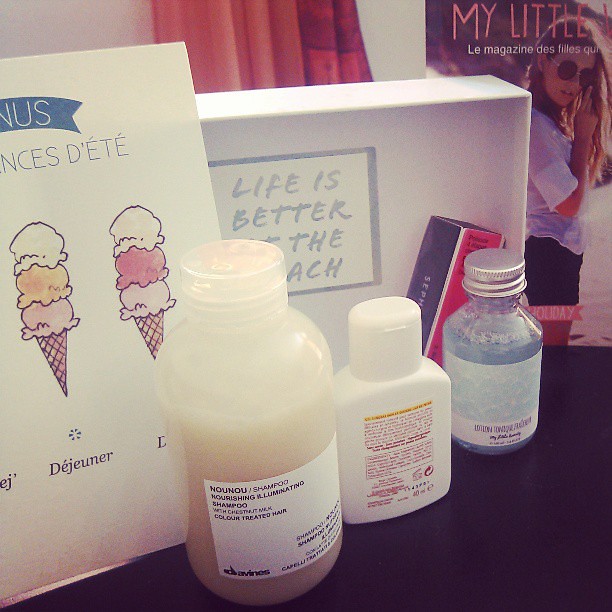The image features three bottles arranged on a dark black surface. The largest bottle on the left is a nearly see-through white plastic bottle with a white label, containing a creamy liquid identified as NuNu shampoo for color-treated hair with chestnut milk. Next to it, there is a flat, rectangular white bottle with a flip-top lid and red writing, although the text is unreadable. The rightmost bottle is a small clear glass bottle with a silver screw-top lid, filled with a bluish liquid, and featuring a white label with the word "lotion" visible. 

In the background, there is a white box standing upright with the text "Life is better at the beach," written in gray-blue letters. Partially obscured behind the bottles is a white card adorned with illustrations of different ice cream scoops and French text. Also visible is part of a poster or magazine that reads "My Little ... Le Magazine des Filles," with an image of a woman wearing sunglasses. The scene is set against a blurry white wall under poor lighting, making the details slightly fuzzy.